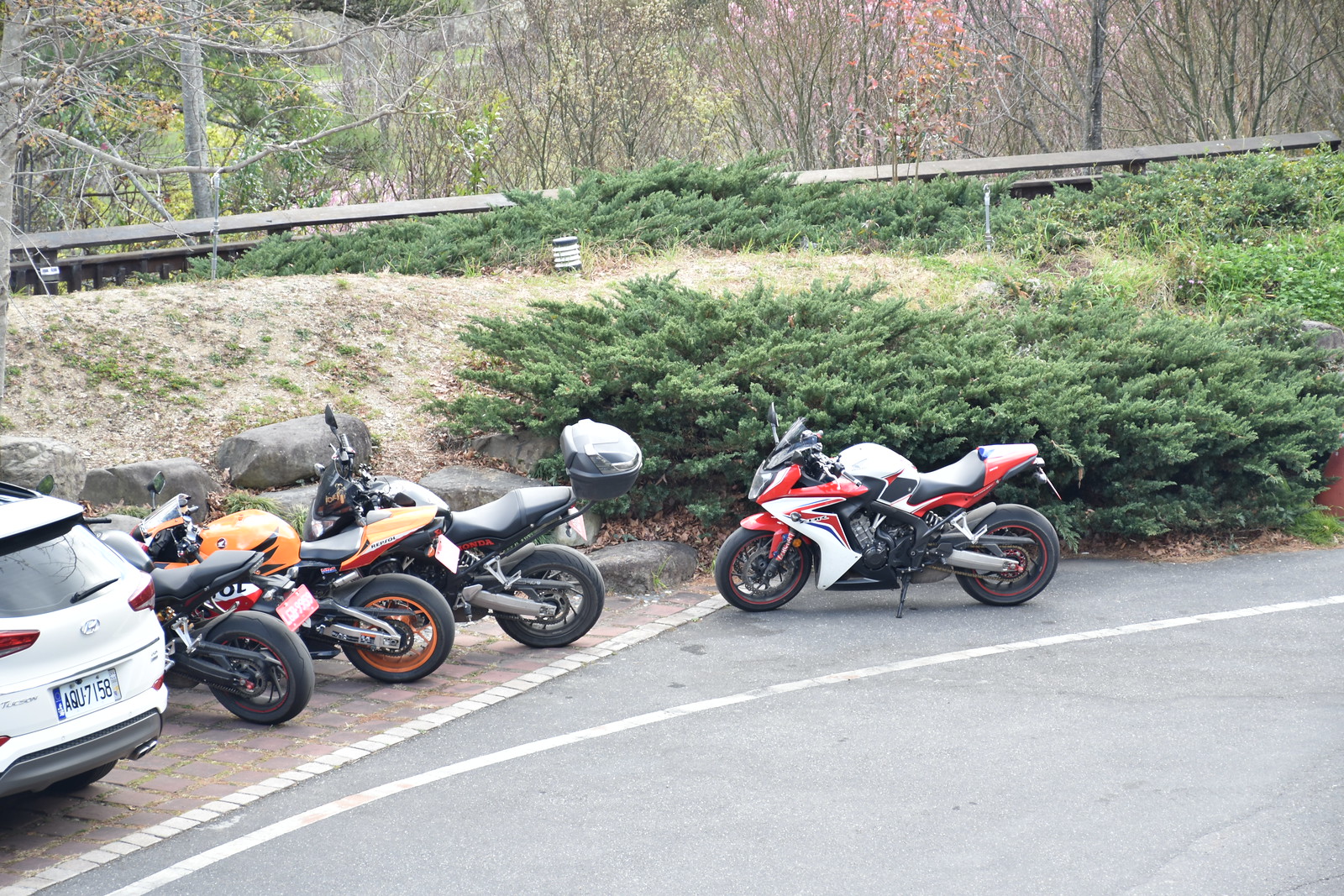This horizontal rectangular photograph captures a corner of a parking lot adjacent to a road. In the bottom left corner, a white hatchback SUV, possibly a Mazda or Hyundai, with a European-style license plate, is parked on a paved concrete area. Directly beside it, three racing-style motorcycles are neatly lined up on what appears to be a cobblestone or brick section of the lot. The motorcycles are yellow, black, and orange and black, with one featuring a gray helmet perched on its back seat. 

Separated slightly from this trio, closer to the lower right corner of the image, a fourth motorcycle stands on asphalt. This bike, characterized by its red, white, and black colors, is positioned further back from the others, with its kickstand down and facing left.

The background of the scene presents a natural landscape, starting with a bushy, low-lying hedge at the edge of the parking area. Behind the hedge rises a small, brown hill adorned with both evergreen bushes and patches of dying grasses. Farther in the distance, a metallic guardrail runs horizontally, aligning with an elevated road or walkway. Beyond the guardrail, several rolling green hills stretch out, dotted with leafless gray-trunked trees, suggesting a late autumn or winter setting. The mix of yellow, red, and green leaves adds a touch of seasonal color to the tranquil backdrop.

Overall, the image vividly details the arrangement of vehicles and the serene, slightly barren landscape framing this secluded parking corner.